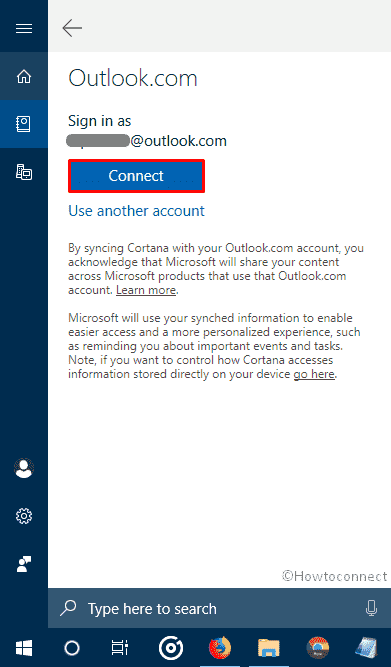In this image from Outlook.com, the interface displays a vertical navigation menu on the left-hand side, featuring a dark blue background. At the top of the menu are three stacked horizontal white lines, often referred to as a hamburger icon. Directly below this icon is a home icon. Further down, we see a section that appears to be selected, depicted by a white background area. This section is marked by an icon resembling a closed book binder. Beneath this selected item, there is an icon that looks like a combination of a PC and a cell phone.

To the right of this vertical menu, the main window prominently displays the Outlook.com logo at the top. Below the logo, it reads "Sign in as," followed by an email address that has been redacted except for the domain "@outlook.com". Underneath this line, there is a "Kinect" button, which stands out due to a red box highlighting it. Following this button, the text "Use another account" is presented, accompanied by two paragraphs that provide information on syncing Cortana with your Outlook.com account. The overall layout and highlighted elements suggest the interface is guiding the user through selecting or managing their accounts and services within Outlook.com.